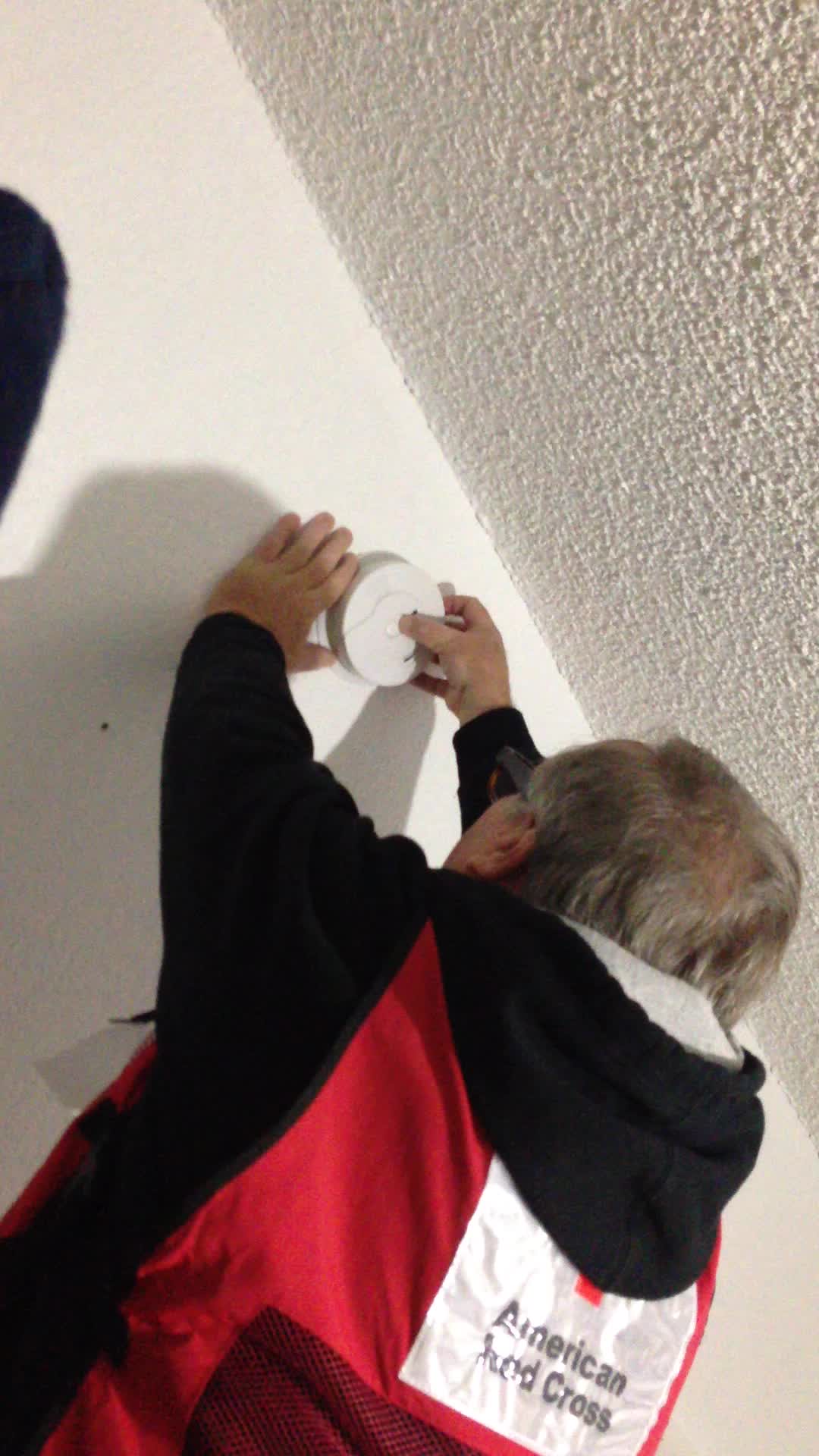In the image, an older Caucasian man with gray hair and glasses is standing near a white, textured wall and ceiling, reaching up high to test or install a smoke detector. He's wearing a distinctive red and black jacket, featuring an American Red Cross logo on the back with a black mesh panel underneath. Both the wall and ceiling are white, with the ceiling more textured, highlighting the man's close proximity to it. The man’s hands are positioned around the circular smoke detector as he pushes the button in the middle, ensuring it is either mounted correctly or functioning properly.